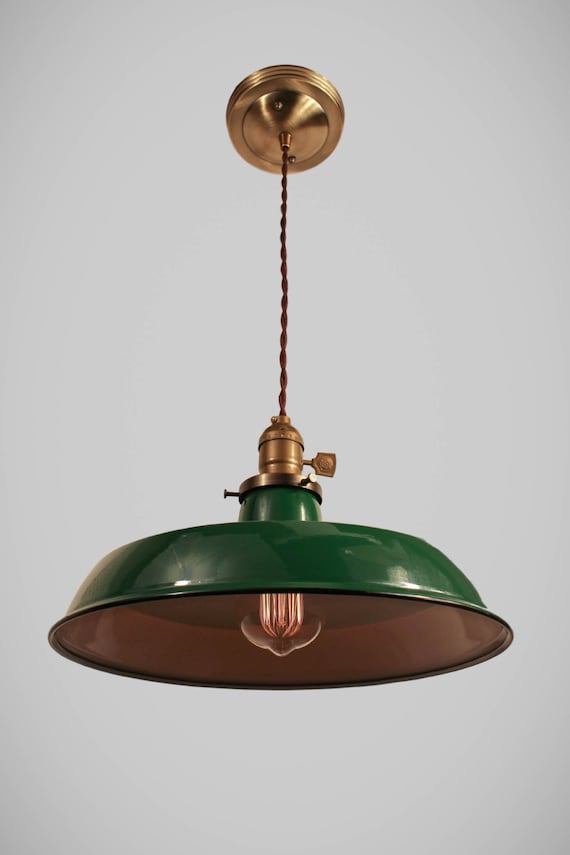This photograph captures a vintage hanging lamp set against a light gray background, suggesting it is attached to a ceiling. The base of the lamp, affixed to the ceiling, is a brass or bronze color from which a twisted, brass-colored cord descends. The cord connects to a brass cone-like fixture that features a brass handle and extends into a broader brass ring with two protruding knobs. The central element of the lamp is a dark green, inverted dish-like lampshade with a bulbous top that flattens out, covering the bulb. The inner surface of the lampshade exhibits a gradient from dark orange to gray. At its core, a light bulb is partially visible, emitting a faint white light and revealing orange vertical filaments within. The lamp's classic design elements, including a nearby brass switch and visible screws, add to its antique appearance and suggest it may be an older fixture, historically rooted rather than contemporary.